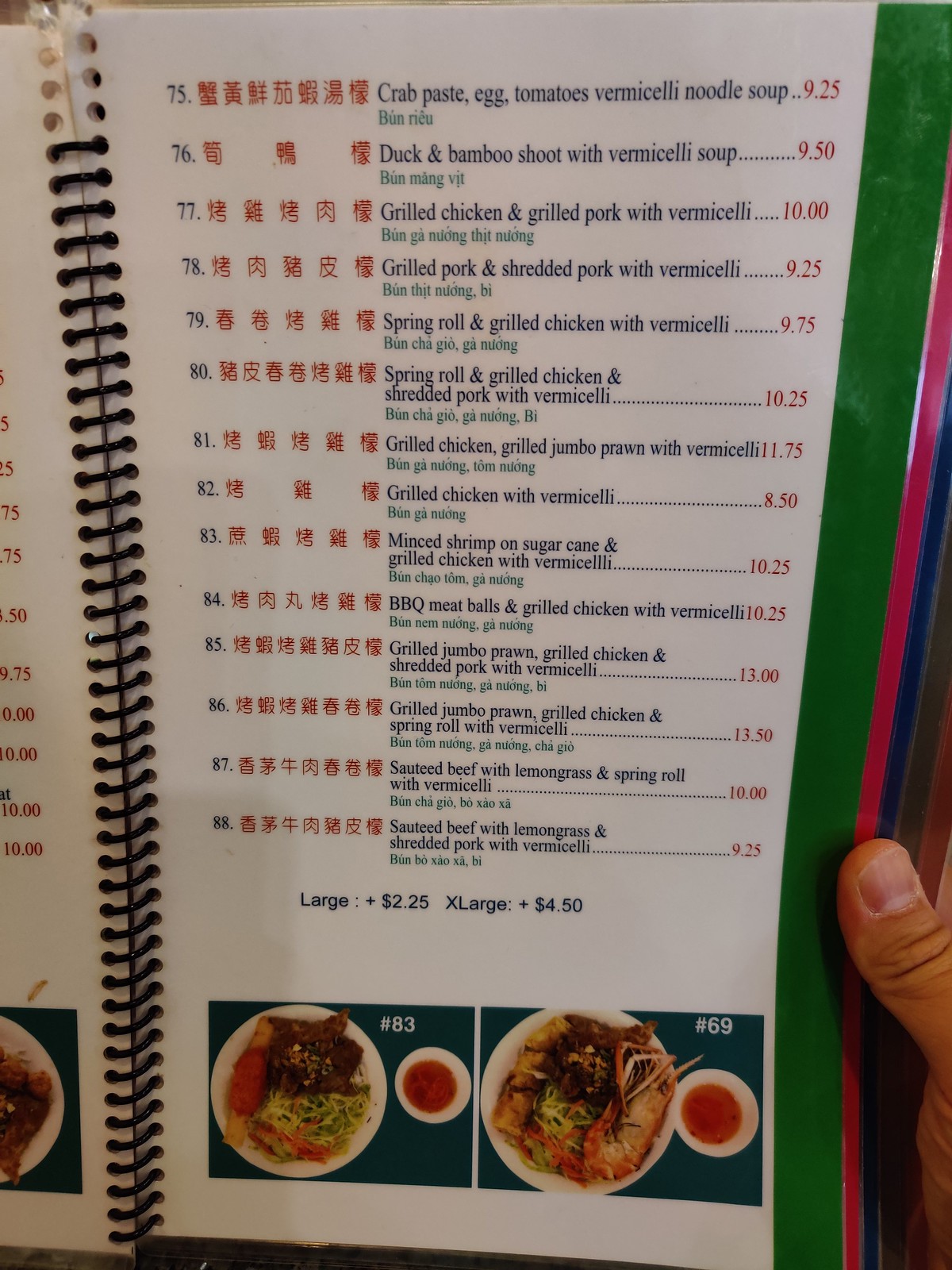The image captures a close-up view of a menu, held up by an individual whose finger is visible in the frame. The menu is aesthetically designed with a green and white background, featuring a red trim along a vertical red strip on the edge. The text is bilingual, comprising of both English and a foreign language with distinct red characters.

Highlighted menu items include:
- Item 75: Crab paste, egg, tomatoes, vermicelli noodle soup priced at $9.25
- Item 76: Duck and bamboo shoots with vermicelli soup priced at $9.50
- Item 77: Grilled chicken and grilled pork with vermicelli priced at $10.78
- A subsequent item of grilled pork and shredded pork with vermicelli priced at $9.25

The detailed layout and bilingual description suggest an inviting and culturally rich dining experience.